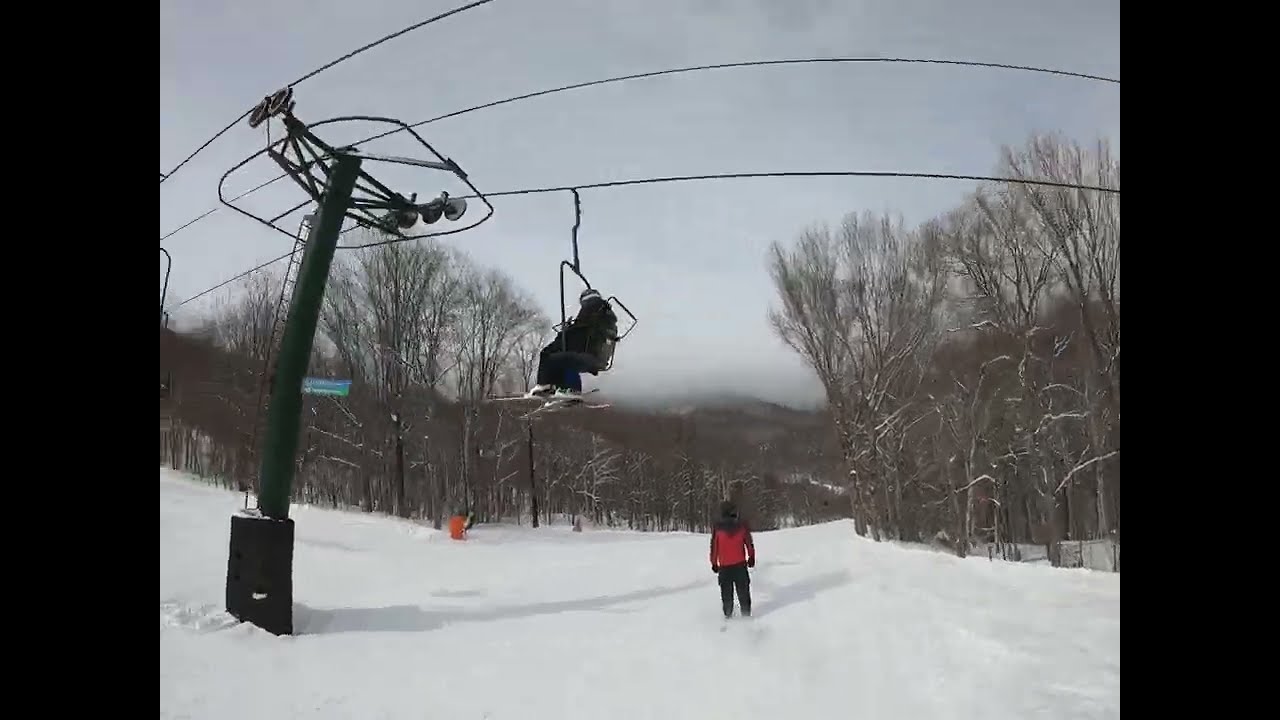The image depicts a snowy winter scene of a ski lift operating at a ski resort. The central focus is a ski lift moving horizontally from right to left, supported by black pillars. A lone skier dressed in a black jacket and pants, with white boots and skis, sits on the lift. Below the lift chair is another person standing on white skis, clad in black pants, a red and black jacket, and a black hat. The ground is covered in a thick layer of snow. Surrounding the ski lift is a small forest of leafless trees, adding to the stark, wintry atmosphere. In the distance, multiple mountains and hills rise under a gray, overcast sky, which casts a dreary, foggy light over the entire scene. To the left of the standing skier, there's an indistinct orange shape—possibly a fallen skier or an orange marker. The image is framed with vertical black borders on the left and right sides, adding to the composed, yet bleak winter landscape.